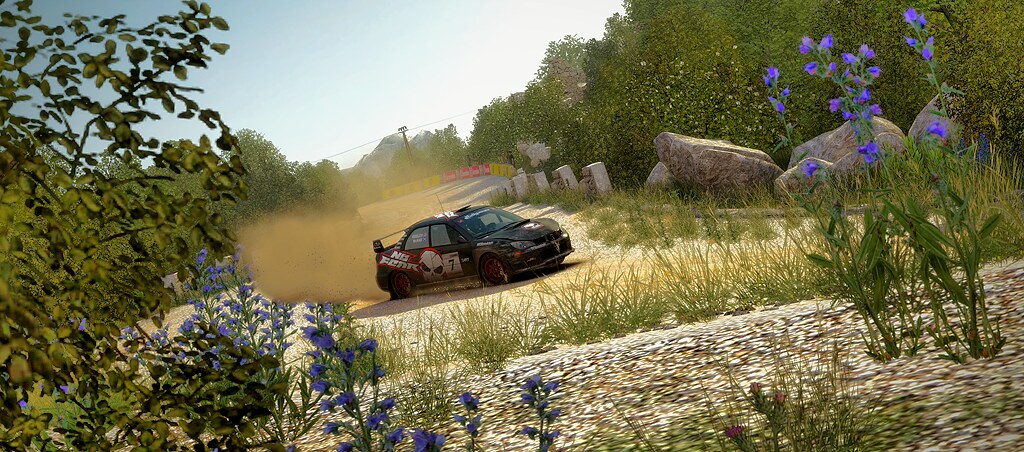In this highly detailed, almost photograph-like still from a video game, the foreground showcases lush green plants interspersed with vibrant purple flowers. The background reveals a landscape of leafy green trees and mountains under a clear blue sky. The grass, depicted in various shades from light to dark green, adds to the natural beauty of the scene. A dusty road cuts through the middle, featuring a dark green car adorned with a black and white skull decal and accented by red and white font. Scattered gray and white stones add texture to the grassy terrain, completing this picturesque and immersive environment.